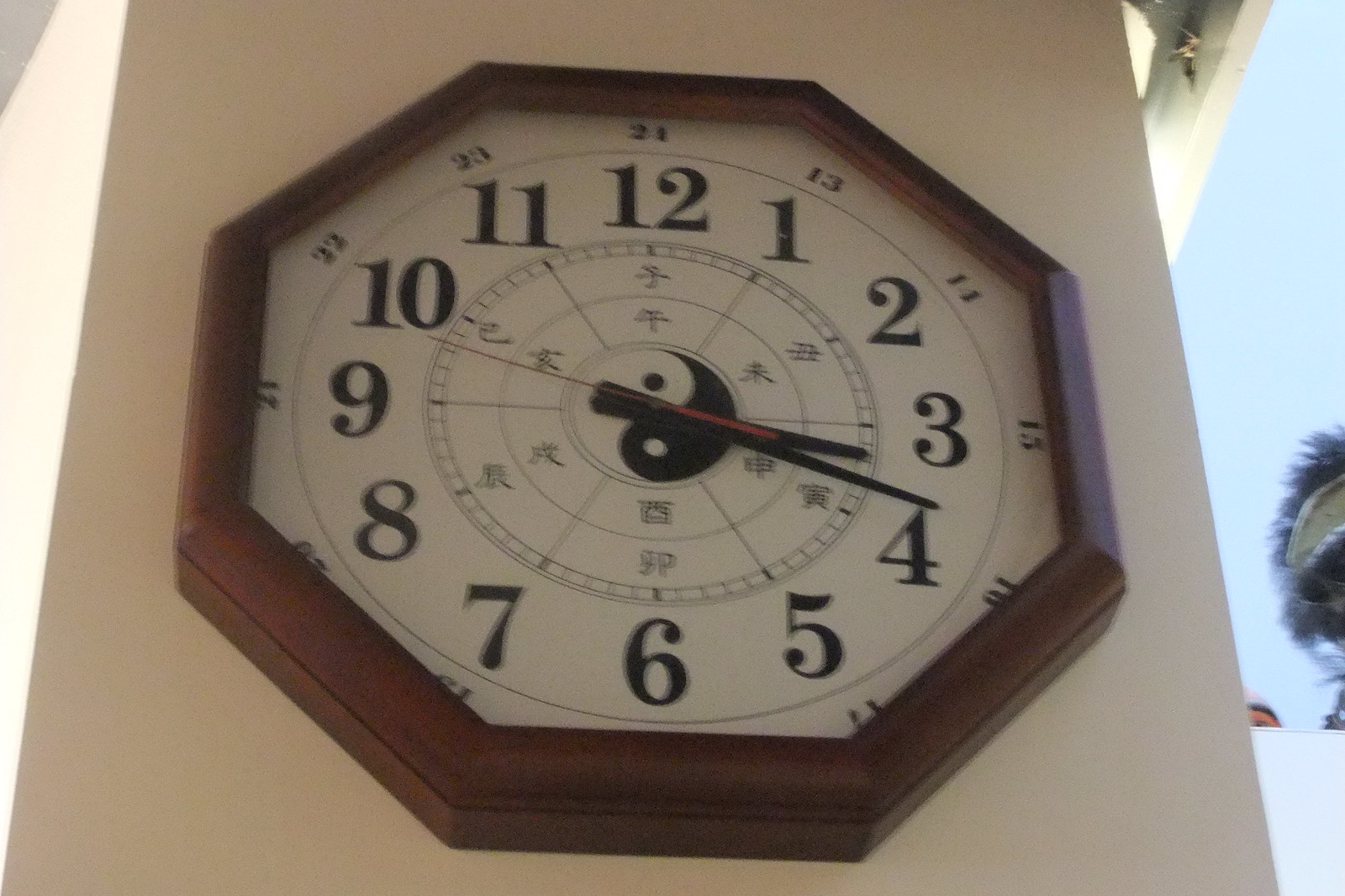The photograph depicts a close-up, low-resolution image of a large, octagonal clock affixed to the exterior of a building with a concrete or stucco facade. The clock is framed by dark, wooden borders and features a unique design. Inside the octagonal wooden frame, there is a circular face displaying the hours 1 through 12 in large, clear numerals. At the center of the clock, a prominent yin-yang symbol is surrounded by traditional Chinese characters, adding an interesting cultural blend to the clock's design. The clock is further characterized by its minute and hour hands, which indicate the time. A clear blue sky is visible in the background, providing a vivid contrast to the details of the clock and the building's facade.